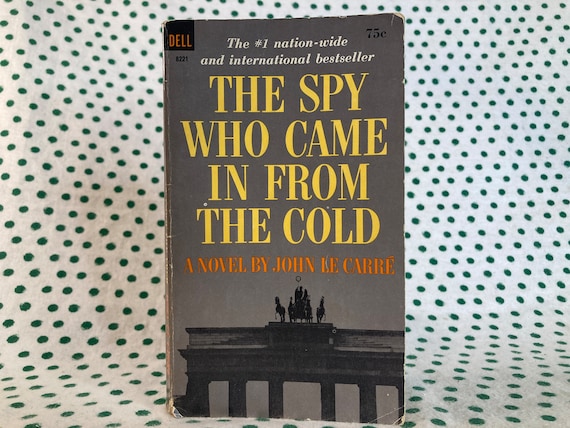This detailed photograph features a vintage paperback book displayed on a polka-dotted piece of fabric, white with green or blue dots. The paperback's gray cover prominently showcases its age with a price of 75 cents printed in the upper right corner. In the upper left corner, the Dell Publishing logo marks the publisher. The title, "The Spy Who Came In From the Cold," stands out in bold yellow lettering, accompanied by white text proclaiming it as "the number one nationwide and international bestseller." Below the title, in amber or orange letters, it reads "a novel by John Le Carré." At the bottom of the cover, there's a black and white photograph depicting what resembles a building's rooftop, possibly adorned with statuary or ornamentation featuring horses, although the exact imagery is somewhat ambiguous. This scene evocatively sets the tone of a cherished classic displayed thoughtfully on patterned cloth.